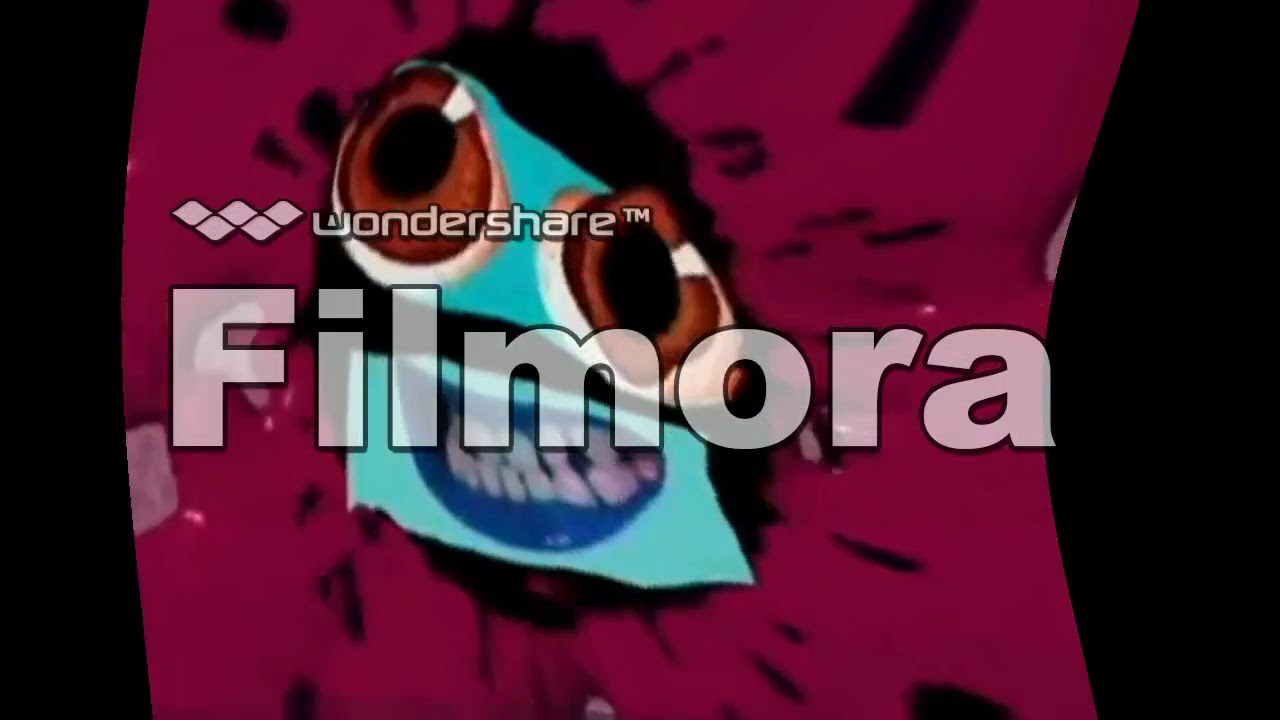The graphic design featured in this image appears to be proprietary, likely an introductory visual for a PowerPoint presentation. Central to the image is a prominent title that reads "Filmora" in large, bold white letters, situated below a smaller watermark that includes the "Wondershare" logo and a trademark symbol. The background consists of a distorted rectangle with a purplish or raspberry hue, bordered by a stark black color. Within this rectangle, a cartoonish face is depicted with exaggerated, expressive features. The face has large brown eyes set against black sclera, and a blue mouth showcasing white teeth. Turquoise stripes and black splatter patterns add a whimsical yet edgy feel to the overall design.